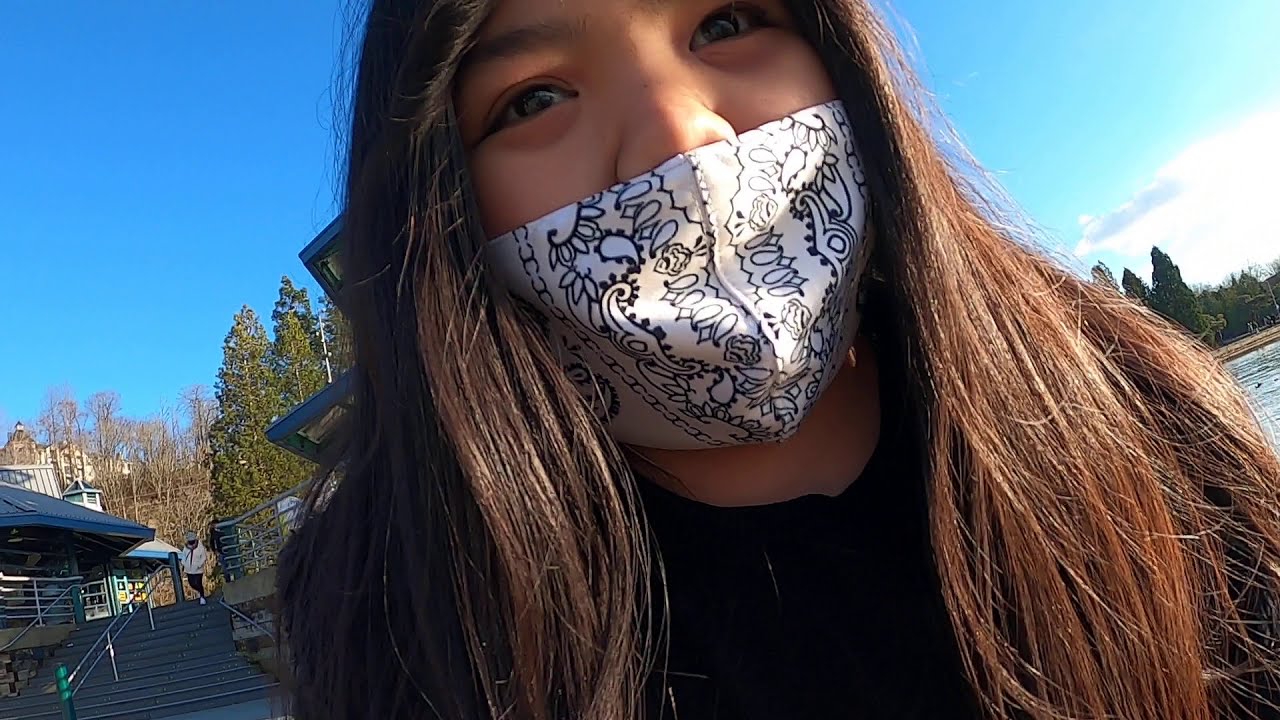The image features a young woman, likely in her late teens, with long, dark brown hair that cascades past her shoulders, some strands catching the sunlight and appearing lighter on the right side. She has dark brown eyes and brown eyebrows, with her face partially covered by a black and white paisley-patterned face mask that conceals her nostrils but not the top of her nose. She is wearing a black top and is gazing upwards, possibly towards the person taking the photo. The background reveals a serene outdoor setting with trees, both deciduous and evergreen, under a partly cloudy, blue sky. To the right, there’s a glimpse of a body of water with a sandbar at the edge. On the left, a concrete stairwell with a handrail is visible, leading to another level where a woman in a white coat is descending the steps. The picture captures a clear day with the sun peeking through the clouds on the right.